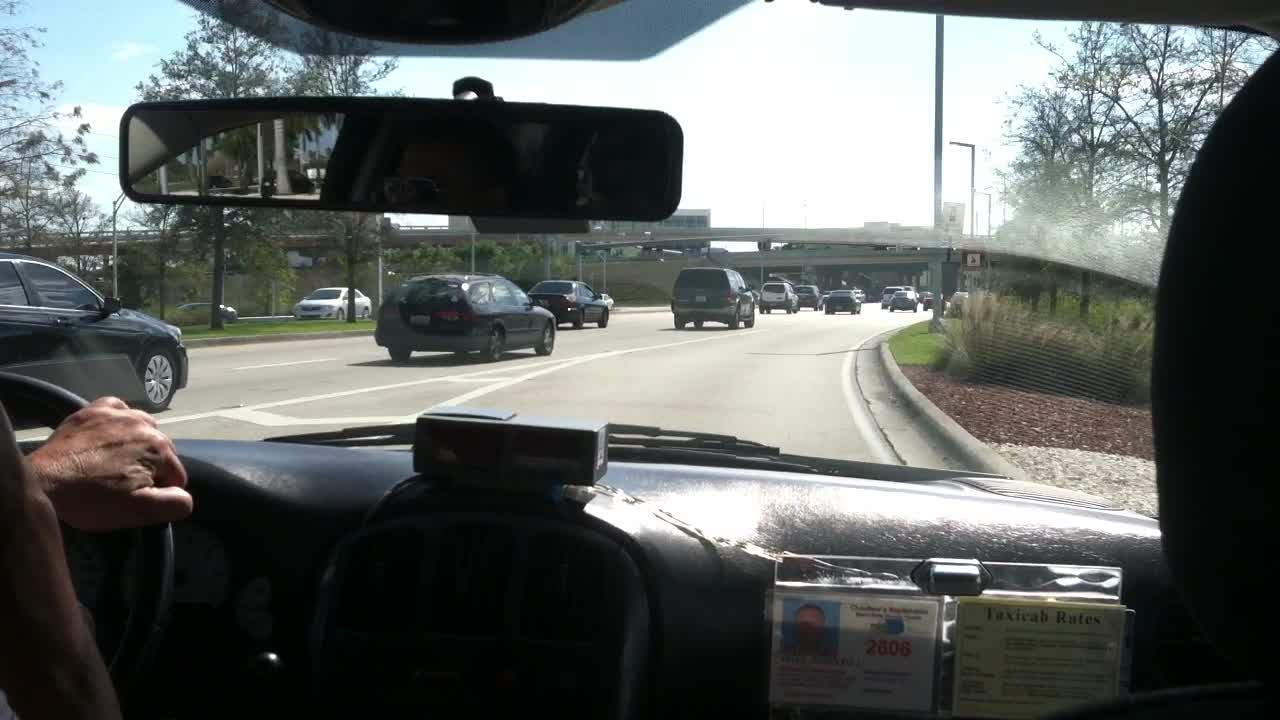This detailed photograph captures the interior of a taxi cab in motion, presumably taken from the backseat by a passenger. The photo prominently features the driver’s left hand on the steering wheel, with a glimpse of his right wrist and forearm visible, indicating his hand is up. The male driver, donning aviator sunglasses and with brown hair, is partially visible through the rearview mirror. The dashboard, with a black plastic finish, displays a cab fare machine, the driver's ID card with a photo and numbers, and a posted taxi cab rates sheet. The scene outside reveals a bright and sunny day as the taxi merges from a ramp onto a moderately busy freeway. The traffic ahead is not bumper-to-bumper but congested enough, with an overpass visible about half a mile away and trees lining the median and sides of the road.